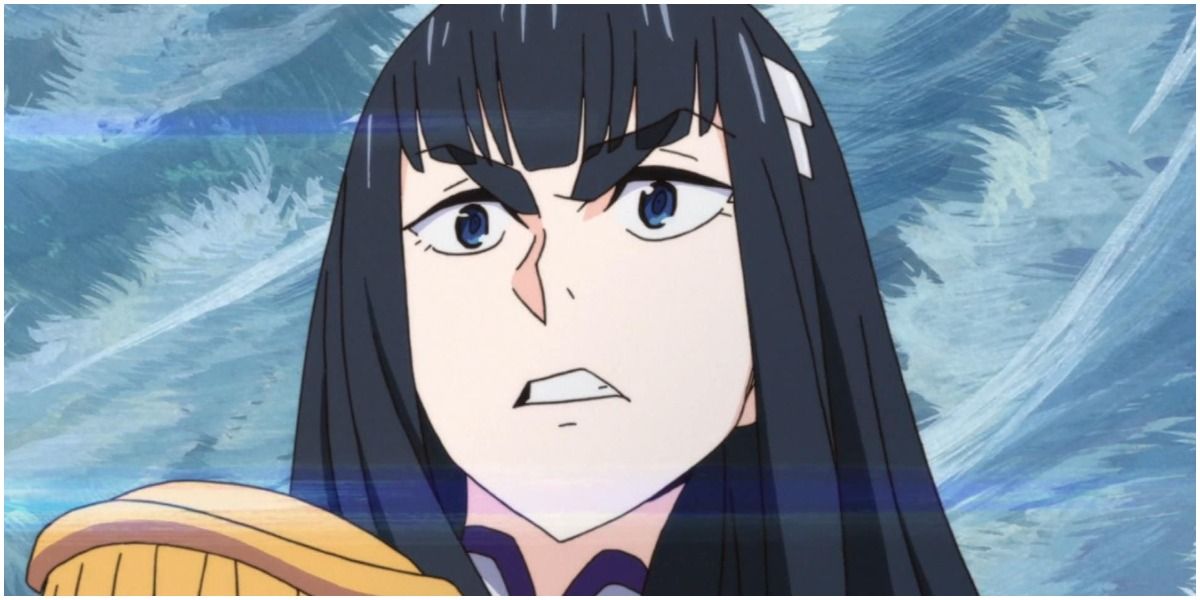This detailed cartoon image features a frightened anime character with large blue eyes and long, straight black hair, accentuated by bangs. A nude-colored barrette clips her hair on the side of her head. She wears a mustard-colored collared shirt, visible only from the shoulders up, with a distinguishable yellow shoulder pad. Her mouth is slightly open, displaying white teeth, and there is pink shading down her nose, highlighting her distressed expression. The background is filled with blue and white feather-like strokes, creating an ethereal atmosphere. This image appears to resemble a film cell from a Japanese manga or anime, complete with blue markings that suggest it captures a fleeting second of animation.